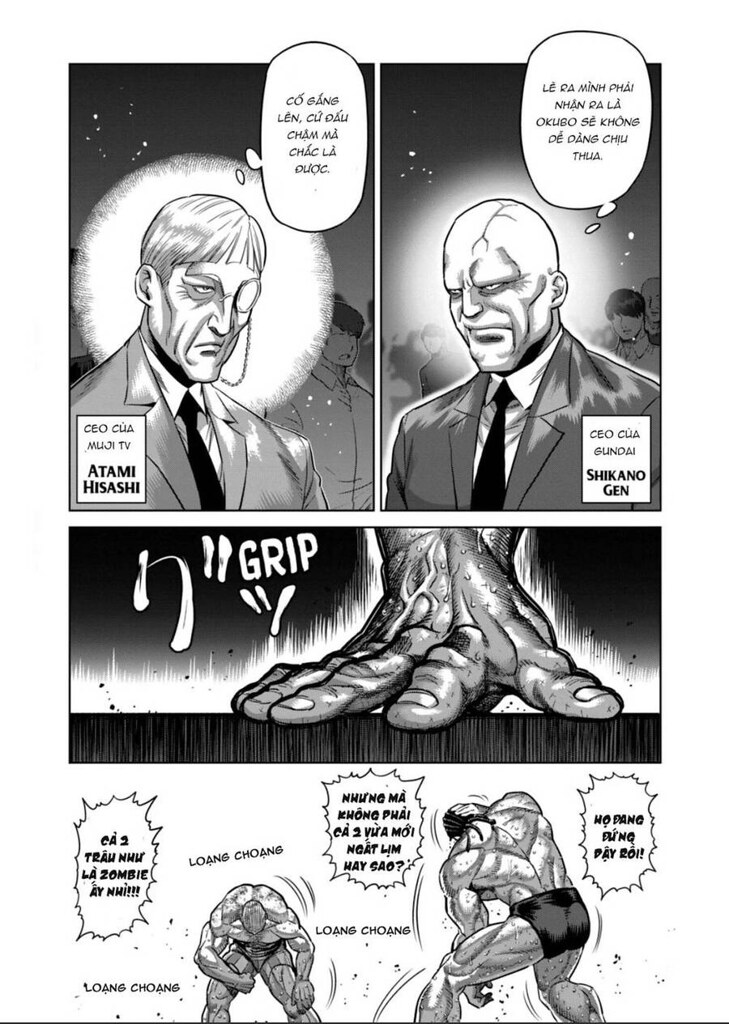The image depicts a captivating comic book scene written in an unfamiliar language, possibly Asian. The narrative seems to involve two distinct characters — one with a peculiar haircut and another, bald with a noticeable scar on his head. Initially, they are depicted as doctors or scientists engaged in what appears to be a serious conversation. This setting quickly transitions into a dramatic transformation; in the middle panel, one character's hand enlarges, mimicking the iconic transformation into the Hulk, with an emphasis on the word "grip." The transformation culminates with both characters morphing into formidable, muscular wrestlers locked in a wrestling match, adding an intense and fantastical twist to the storyline.